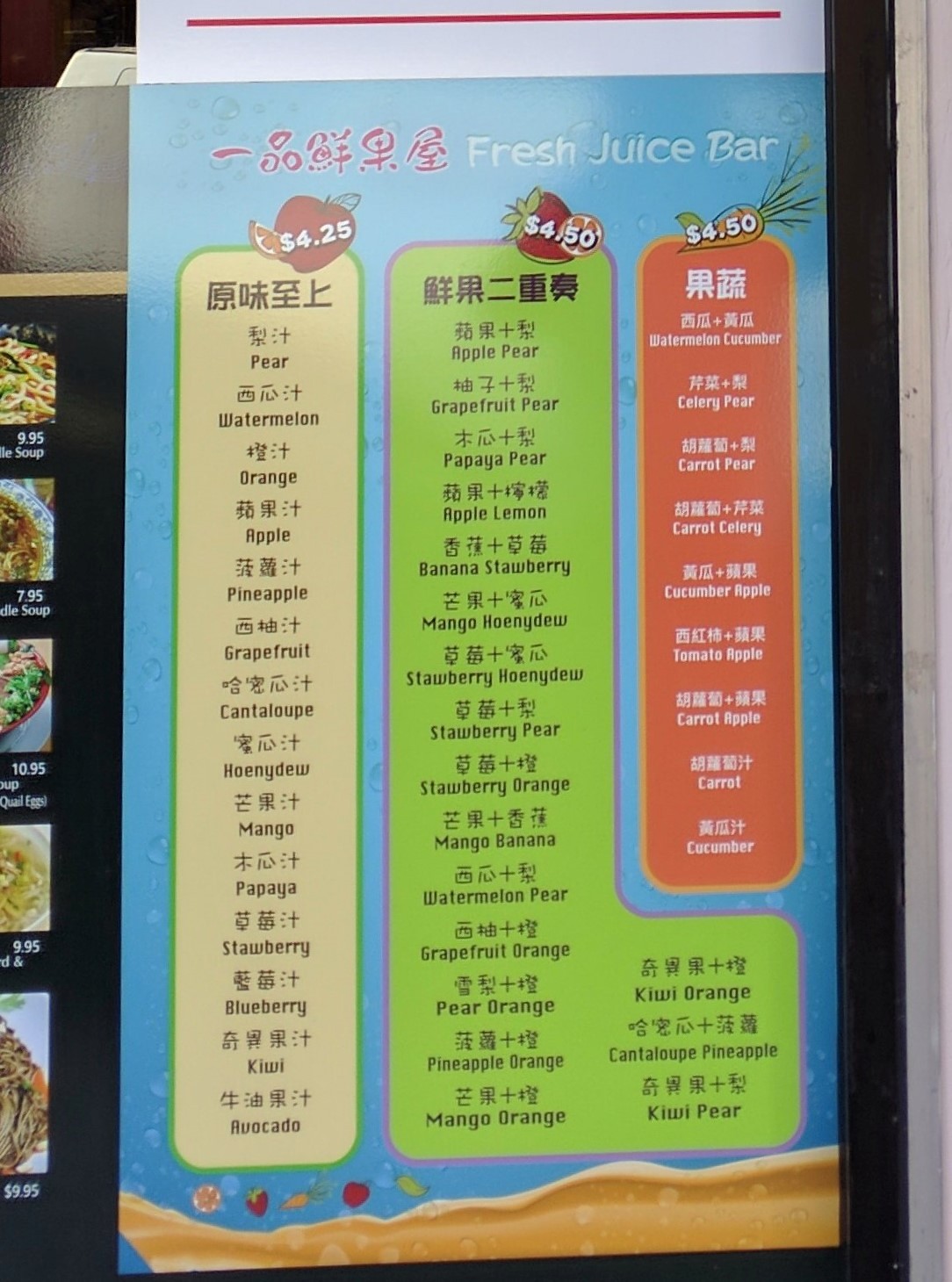This photograph, captured in portrait mode, offers a close-up of a menu tucked behind a mottled, water-streaked glass. The upper portion of the menu features a distinctive white strip with a red line running horizontally from the upper left to the upper right corner. The glass covering the menu is blurred and appears wet, obscuring the details beneath.

The menu itself includes three distinct columns prominently displaying various beverage options. The first column features a long yellow oval outlined in green listing various fruit juices: pear, watermelon, orange, apple, pineapple, grapefruit, cantaloupe, honeydew (misspelled as "honey dew"), mango, papaya, strawberry, blueberry, kiwi, and avocado. Small illustrations of strawberries and carrots accompany these listings, with a price of $4.25 prominently displayed above an image of a strawberry and orange.

The second column is notably wider, featuring a light green background framed in purple. It lists an assortment of juice combinations: apple-pear, grapefruit-pear, papaya-pear, apple-lemon, banana-strawberry, mango-honeydew (misspelled), strawberry-honeydew (misspelled), strawberry-pear, strawberry-orange, mango-banana, watermelon-pear, grapefruit-orange, pear-orange, pineapple-orange, and mango-orange. This column is priced at $4.50, with images of a strawberry and an orange positioned at the top for visual reference. Near the bottom, the text extends rightward in a list shaped like an L, including kiwi-orange, cantaloupe-pineapple, and kiwi-pear combinations.

The third column, against a bold orange background outlined in light orange, lists vegetable and fruit mixes at $4.50. It includes watermelon-cucumber, celery-pear, carrot-pear, carrot-celery, cucumber-apple, tomato-apple, carrot-apple, carrot-cucumber, and apple combinations, all framed by a blue backdrop.

In the lower left section of the image, a black background features five partial photographs of the establishment’s food offerings, accompanied by their prices: $9.95 for soup, $7.95 for another soup option, $10.95 for a quail egg soup, and two more dishes each priced at $9.95. These images provide a glimpse of the diverse menu items available to customers.